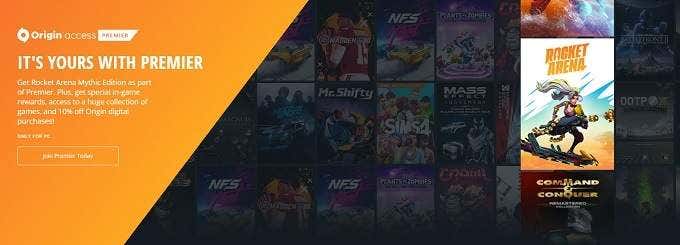The image features a screen from a movie-related site, with a sleek and visually engaging design. Dominating the top left corner is the bold text "Origin Access Premier," under which the phrase "It's Yours with Premier" is prominently displayed in white. Beneath this header lies a paragraph in white text, though its content is not specified. Just below the paragraph, a conspicuous call-to-action button reads "Join Premier Today" within a clearly defined rectangle.

The leftmost 30% of the image is shaped like a trapezoid, creating a distinct division between the vibrant orange background on the left and the dynamic holographic black background on the right. This separation is marked by a slanted line, contributing to the image's modern and edgy aesthetic.

On the right side, the holographic black background hosts the main content: three rows of movie title listings. One title stands out, highlighted for selection: "Rocket Arena," displayed in striking orange text. Adjacent to this title is an eye-catching logo depicting a character engaged in what appears to be playing a guitar while riding a snowboard. This logo is predominantly black with an orange base, interspersed with blue designs behind the character, and capped with a white top.

Directly below "Rocket Arena," the classic title "Command and Conquer" is listed against a dark brown background, rounding out the image with a sense of nostalgia and excitement. The overall composition effectively blends colors and shapes to create an engaging and informative visual experience.